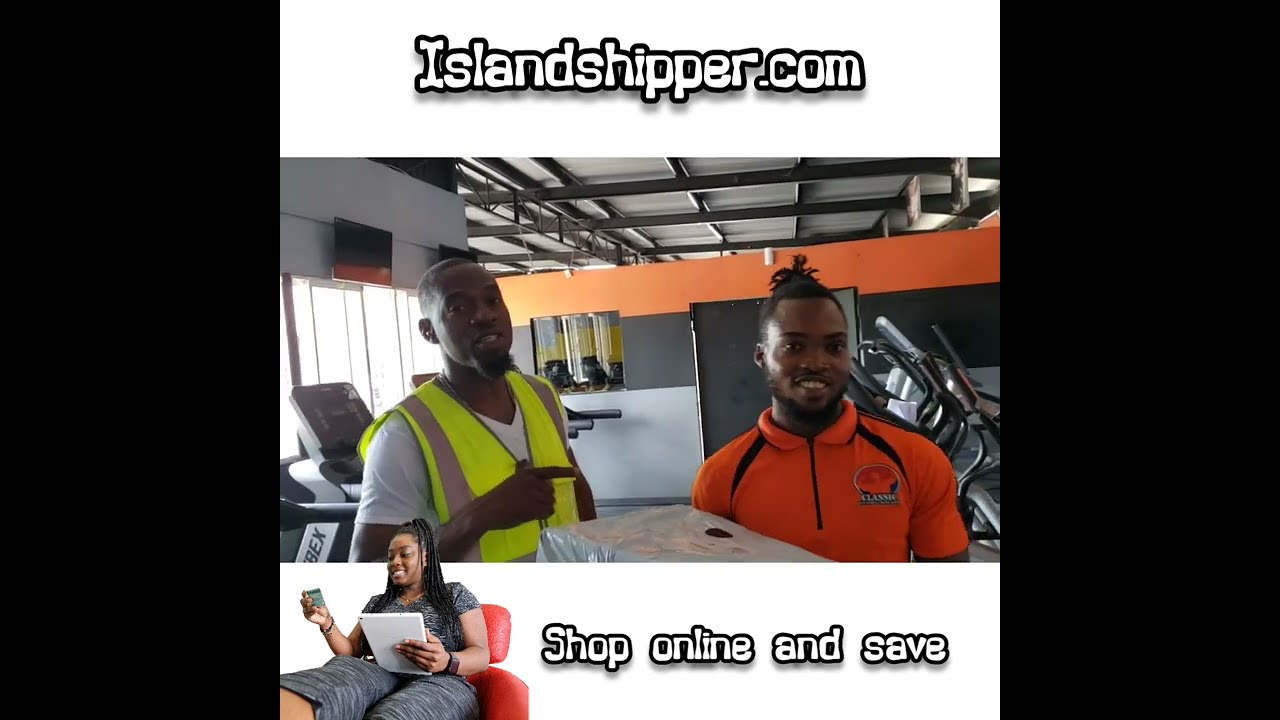This image appears to be a poster or advertisement for "islandshipper.com," prominently displayed in white font with a black outline at the top. The poster features two young African-American men in their 20s, likely delivery personnel, standing in a room that resembles a fitness facility, identifiable by gym equipment like treadmills and cycle machines in the background. 

The man on the left is partially obscured but is wearing a yellow fluorescent safety vest with silver stripes, a white V-neck t-shirt, and has a thin black goatee. He points towards the man on the right, who is more clearly visible, sporting an orange short-sleeved polo shirt with a zipper and black detailing. This man has his hair styled in tied-up dreadlocks and wears a thin black beard and mustache. Both men are smiling and holding a white package wrapped in plastic, indicative of their delivery roles.

In the lower part of the poster, the text "shop online and save" appears in the same white and black-outlined font. To the left of this text is an image of an African-American woman sitting in a red chair, dressed in a gray outfit with a white stripe. She holds a credit card in one hand and a tablet in the other, further emphasizing the online shopping theme. The background also features a gray-tile ceiling with black metal beams and sunlight streaming through windows.